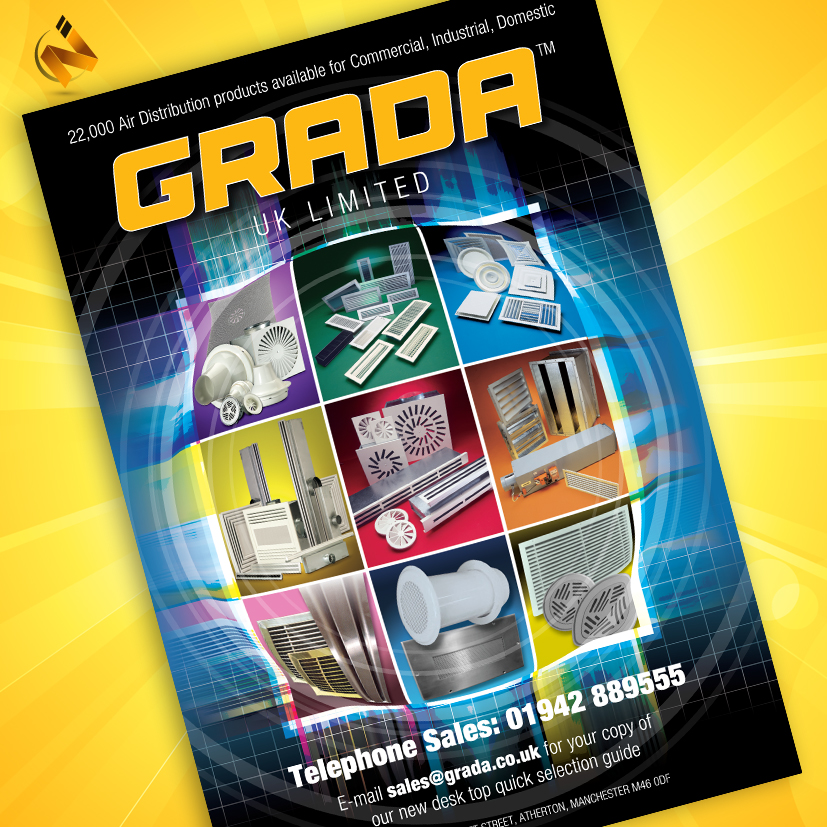The image is a digitally generated flyer for Grada UK Limited, showcasing their extensive catalog on a yellow background. The catalog cover is positioned diagonally with the top and bottom sections in black and the central part featuring a circular design with shades of blue and multiple colored segments. These segments form a circle divided into nine equal parts, each depicting various air distribution products such as exhaust fans, air conditioners, and vents. At the top of the flyer, the text in white font reads "22,000 air distribution products available for commercial, industrial, and domestic." Below this, in yellow font, it says "Grada," followed by "UK Limited" in white. The bottom of the flyer provides contact details: "telephone sales 01942889555" and "email sales at grada.co.uk for your copy of our new desktop quick selection guide" in white font. The background behind the catalog appears to be shining, giving the overall image a vibrant look.